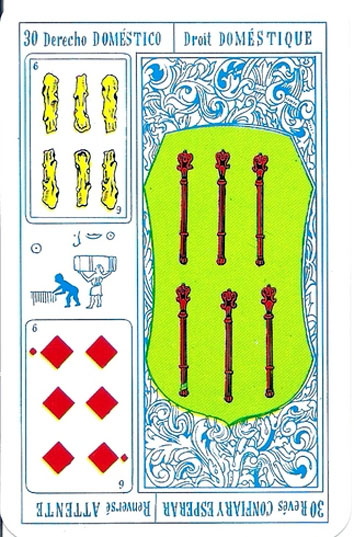### Detailed Descriptive Caption:

The image is an intricately detailed illustration, potentially resembling a card of some sort, with a vertical orientation, being taller than it is wide. The primary color theme features blue lettering and stenciling set against a white background, though elements of other colors are included. 

At the top left corner, in blue, is the text "30 Derecho Doméstico," which translates from Spanish to "30 Domestic Right." Mirroring this, the top right corner presents "Droit Domestique," translating from French to "Domestic Right," albeit the term "right" is misspelled as "R-A-G-H-T."

The illustration is divided into multiple sections. Directly beneath the Spanish text, there's what resembles a tarot card in a subsection, depicting the "Six of Clubs" with the card suit drawn in yellow. Both the top and bottom of this card display the number six.

Continuing downwards on the left side, an Egyptian hieroglyph style illustration is visible. This depicts two figures: one appears to be carrying an object on their shoulder, while the other seems to be bending over, possibly engaging with a plow. Below this hieroglyph is another card section showing the "Six of Diamonds."

Occupying around two-thirds of the card's width on the right-hand side is a depiction of six red clubs set against a blue and white background featuring a blue fleur-de-lis pattern.

At the very bottom of the card, the text mirrors the wording at the top but is presented upside down. The overall composition suggests the significance of the number six, expressed through various stylistic representations.